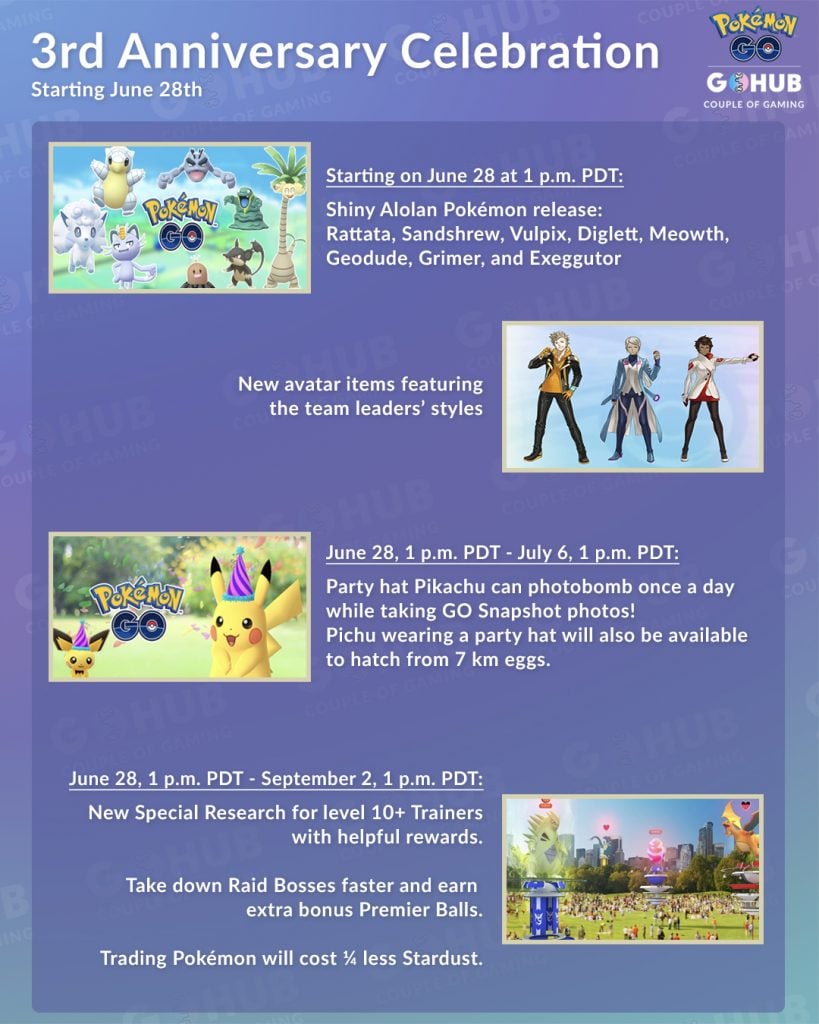The image features a vibrant ombre background transitioning from a light pinkish-purple at the top, descending into a bluish-lilac in the middle, and finally fading into a sea breeze green at the bottom. At the top of the image, "3RD Anniversary Celebration" is prominently displayed in white text. Below that, the event dates are clearly stated as "Starts June 28th."

On the right side of the image, the iconic "Pokémon" logo stands out in its traditional yellow with a blue outline, complete with the accented 'é' and a red and white Poké Ball embedded in the 'o'. Below this logo, the text "GO Hub" is displayed, with the letters transitioning from blue to pink.

Towards the bottom of the image, a darker purple box contains text in white that reads: 
"Starting on June 28th at 1 p.m. PDT
Shiny Alolan Pokémon release:
Rattata, Sandshrew, Vulpix, Diglett, Meowth, Geodude, Grimer, and Exeggutor."

Additionally, the image mentions "New items featuring Team Leaders' style" as part of the celebration.